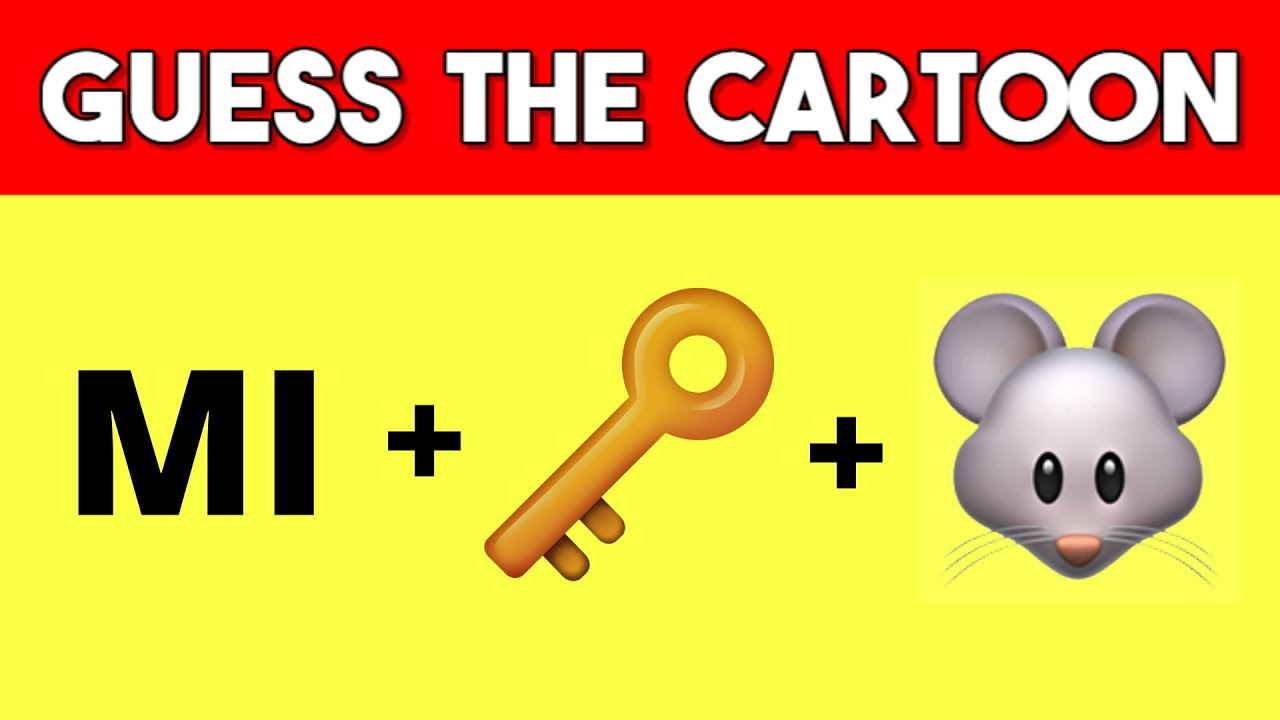This bright and simplistic poster features a large red banner at the top with bold white block letters that read "Guess the Cartoon." Below the banner, the poster is divided into two sections differentiated by color: a large yellow rectangle fills the bottom two-thirds of the image. Within this yellow section, there are black letters spelling out "M.I." followed by a plus sign. Next to the plus sign is a diagonal image of an old-fashioned skeleton key, depicted in a yellowish color. Another black plus sign follows the key, leading to an illustration of a cute gray mouse head. The mouse has round ears, a heart-shaped face with puffed-out cheeks, oval black eyes with white dots, a pink nose, and visible whiskers. The overall design layout is horizontal, and the combination of elements on the poster forms a Rebus puzzle that encourages viewers to guess "Mickey Mouse." The use of bold colors and simple illustrations makes it particularly appealing to young children.